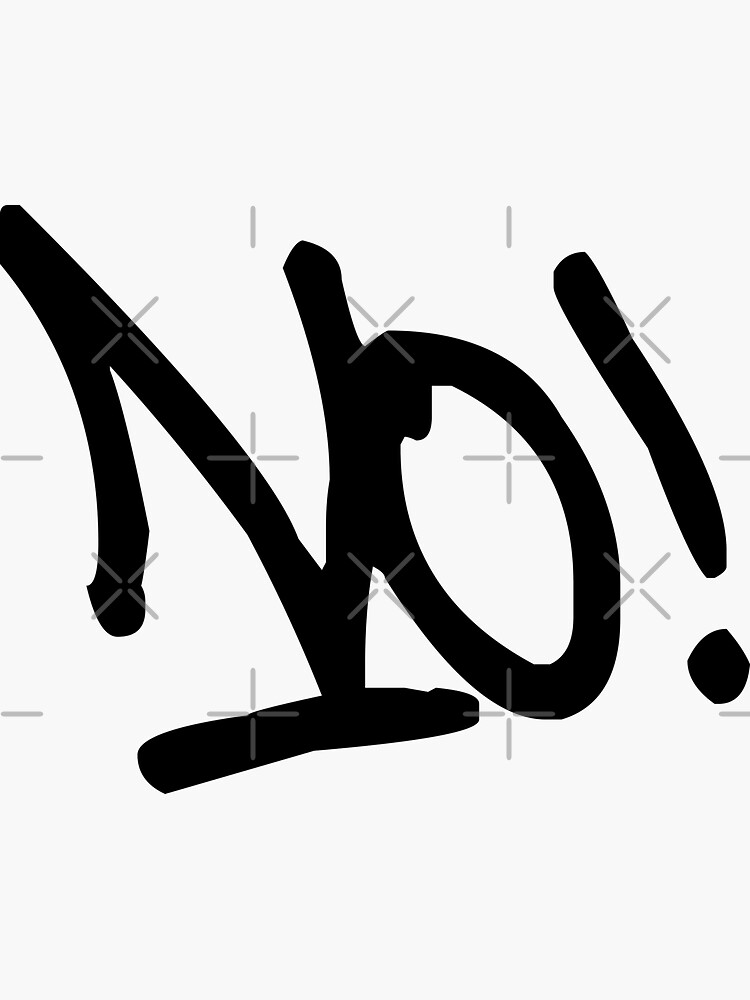This image depicts a digitally created sketch on MS Paint, featuring the word "NO!" in bold, black ink on a white background. The lettering is large and slightly slanted towards the bottom right, with the "N" and "O" joined together dynamically. The word is underlined by a thick horizontal line that intersects two of the three lines of the "N." Beneath the main text, there is a small signature or emblem reading "Stick Aya" in a simple font, located in the bottom right corner. The overall composition is striking and minimalist, clearly designed to emphasize the urgent and imperative nature of the word.